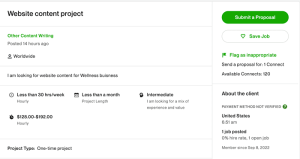This image is a low-quality screenshot of a webpage pertaining to a website content project. The background is white with a light grey grid overlay. The text is predominantly black with some sections highlighted in green.

- **Top Bar**: The top bar reads "Website Content Project."
- **First Section**: This area seems to be titled "Office Centered Writing" and indicates the project was published approximately 14 hours ago and is open to worldwide contributors. It states, "I am looking for website content for [possibly 'website business']."
- **Middle Section**: Further stipulations are provided, but they are difficult to decipher due to the screenshot's poor quality. However, it is noted that the "Project type" is a one-time project.
- **Right-Hand Side**: There are two prominent buttons: "Submit a Proposal" at the top and "Save Job" below it.
- **Additional Options**: Following these buttons, there are more options such as "Flag as Inappropriate," "Send a Proposal," and "Connect." An option or section labeled "Available Comments" is also mentioned but is unreadable.
- **Remainder of Content**: The bottom section of the screenshot is unreadable and lacks discernible details.

This detailed caption aims to give a comprehensive understanding of the contents and structure of the screenshot despite its low resolution.